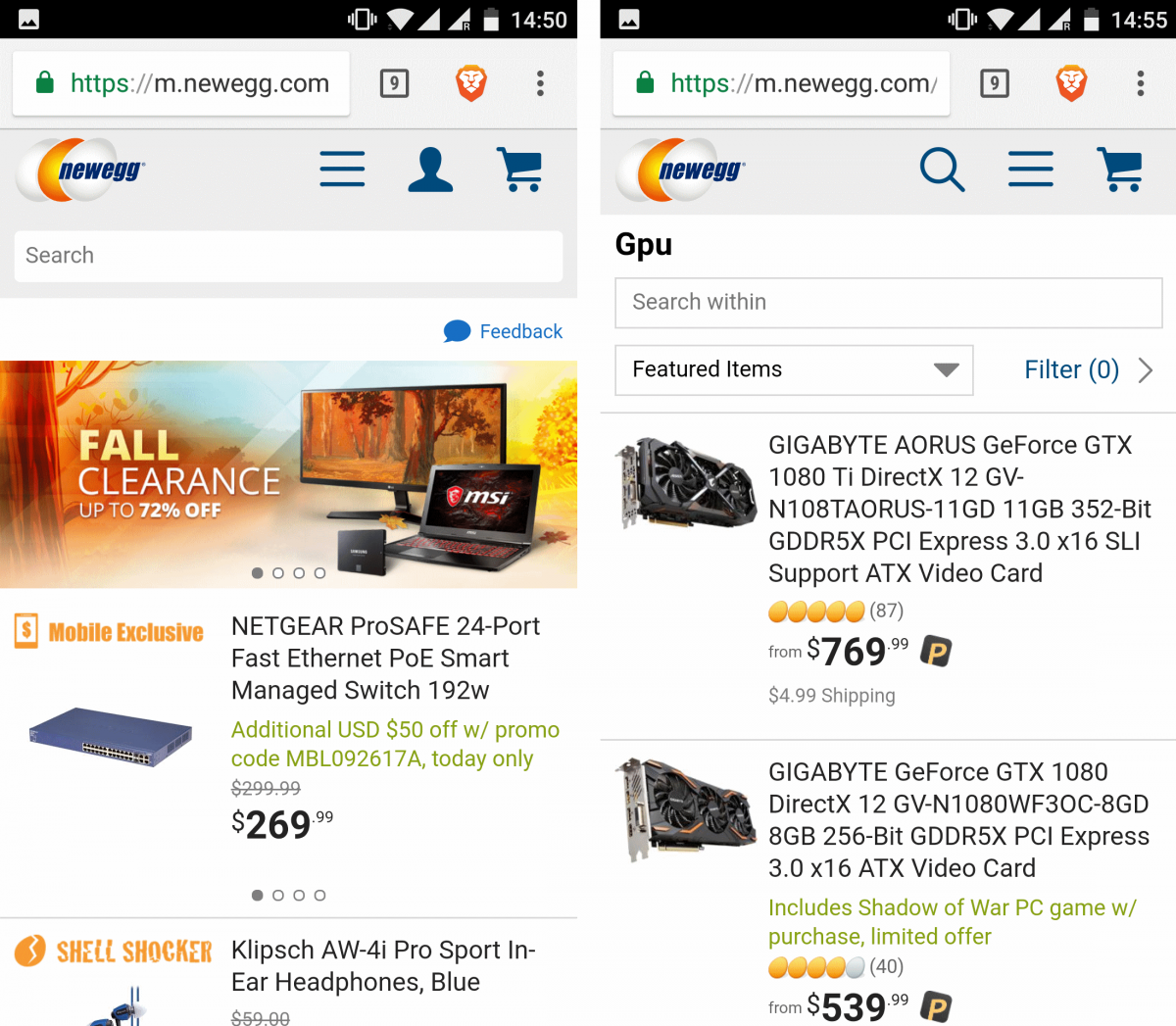On the Newegg mobile site, we see two images displayed side-by-side. The left image showcases what appears to be the homepage, highlighting a "Fall Clearance" sale offering discounts of up to 72%. Prominently featured is a widescreen monitor, an MSI laptop, and a small SSD. In addition, various products are listed, including a Netgear 24-port Fast Ethernet PoE Smart-Managed Switch and Klipsch headphones, though the headphones' price is not visible.

The right image seems to be the result of a search for GPUs (graphics processing units). Two specific GPUs are listed: the first is a Gigabyte Aorus GTX 1080 Ti, priced at $770, with a perfect rating of five eggs out of five. The second GPU is a standard GTX 1080, priced at $540, featuring slightly lower specifications and rated four eggs out of five. This GPU also comes with a limited offer of the Shadow of War PC game. The browser in use appears to be Brave, identifiable by the lion head icon at the top, and there are nine other tabs open in the browser.